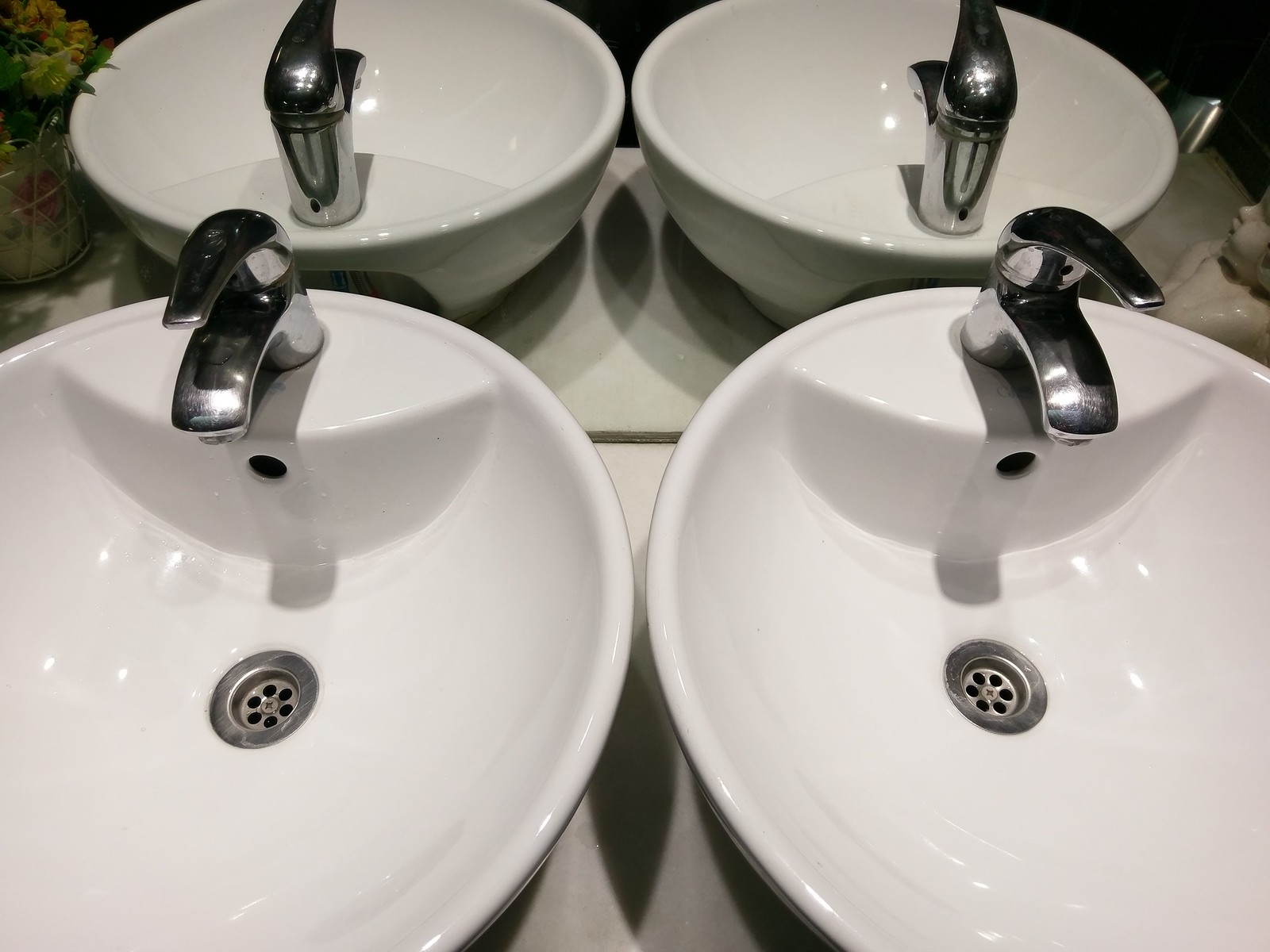The photograph depicts a modern bathroom setup with an intricately designed layout against a white tiled background. At first glance, it shows what appears to be four sinks, but upon closer inspection, it's actually two white, round, porcelain basins whose reflections in a large, wide mirror behind them create the illusion of four. Each basin sits atop a charcoal gray countertop and features sterling silver fixtures, including a lever faucet for adjusting water temperature and a stainless steel-colored drain and switch. The faucets of the front basins face toward the camera, while the reflected faucets of the back basins face away. To the left, the mirror reflects a flowering pot plant, housed in a wrought iron basket. On the far right, perched on the basin's edge, there's a small, off-white ceramic angel or cherub figure, partially visible, adding a whimsical touch to the scene.